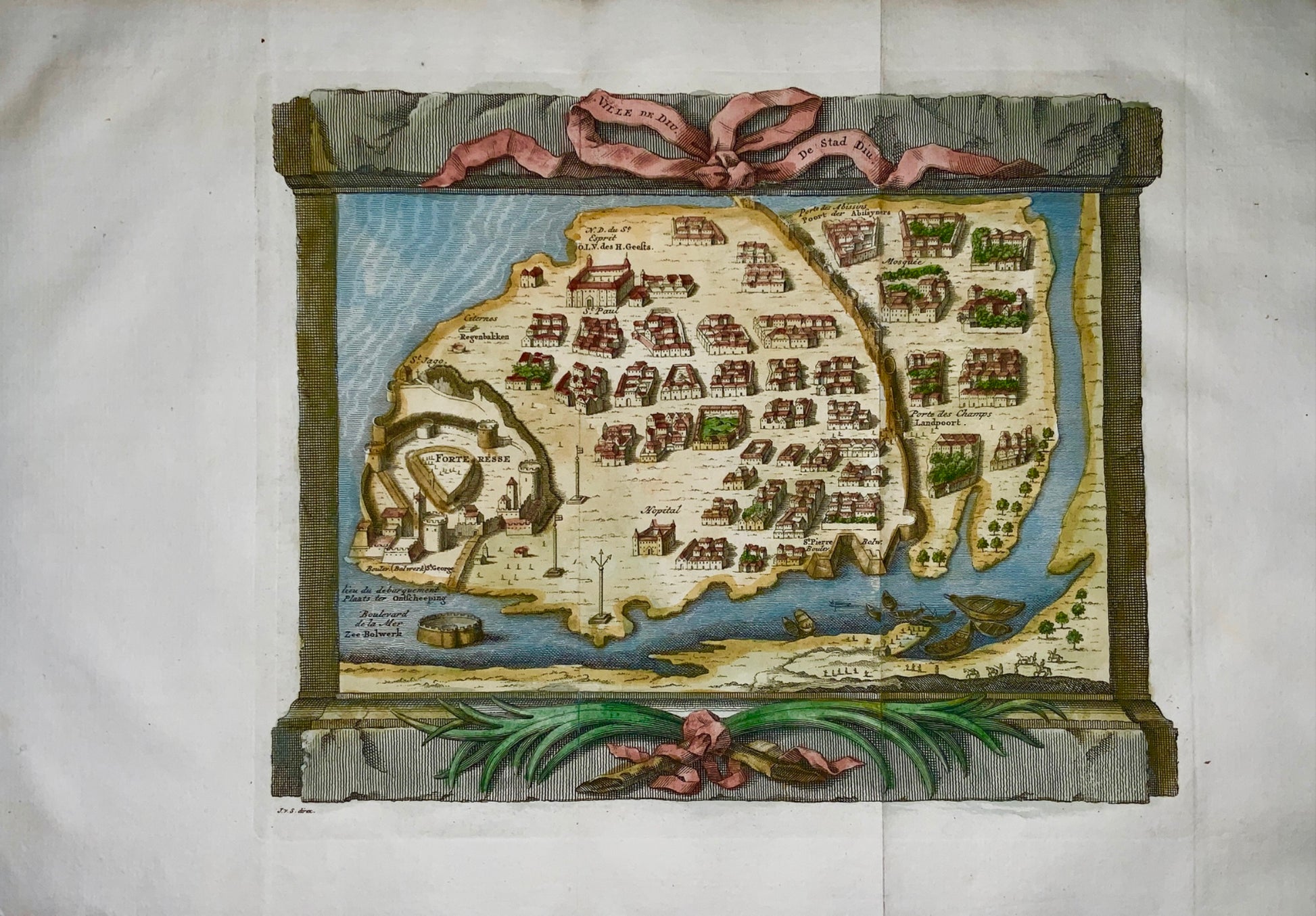The image depicts a detailed, illustrated tapestry crafted to resemble an old-world map of an island, bordered by wooden framework. Both the top and bottom edges of the tapestry are adorned with gray fabric; the top section is further embellished with a red ribbon featuring ornate writing, possibly in a different language, while the bottom part includes a green branch with petals, adding a botanical touch. The centerpiece of the tapestry features a vintage-style map made to look like parchment paper, despite being woven. The map showcases a small town and a fort labeled "Fort Reese" on the left side, numerous small buildings, a possible church, and a large dividing wall on the right. At the bottom left, near the fort, there are three poles that seem to represent flags. Additional details include a fort appearing to be in the water and several boats along the coastline of a nearby larger landmass. The map is rich with various landmarks and is surrounded entirely by water.